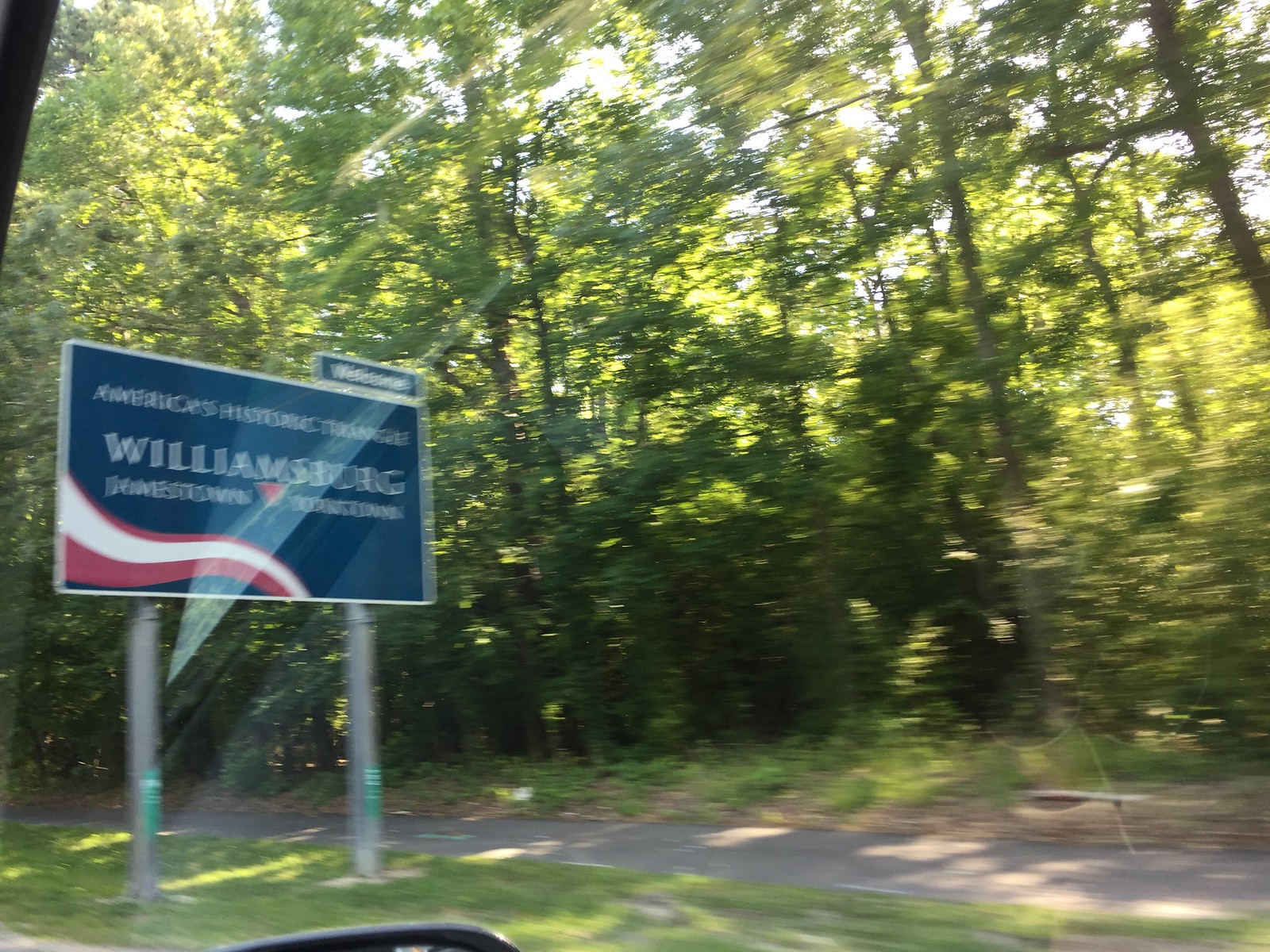This photograph, taken from a moving vehicle, features a noticeable motion blur evident in the trees, indicating the car's speed. The slightly out-of-focus shot captures the top edge of the vehicle's rearview mirror at the bottom of the frame. In the distance, a prominent sign reads, "Williamsburg, Jamestown, Yorktown, America's Historic Triangle, Welcome," adorned with a red and white banner on a deep blue background, supported by silver vertical posts. Sunlight filters gently through the leafy trees, illuminating what appears to be a walking or biking path alongside the road. In the lower right corner, a bench or seating area is faintly visible, suggesting a spot for rest or congregation along the pathway.